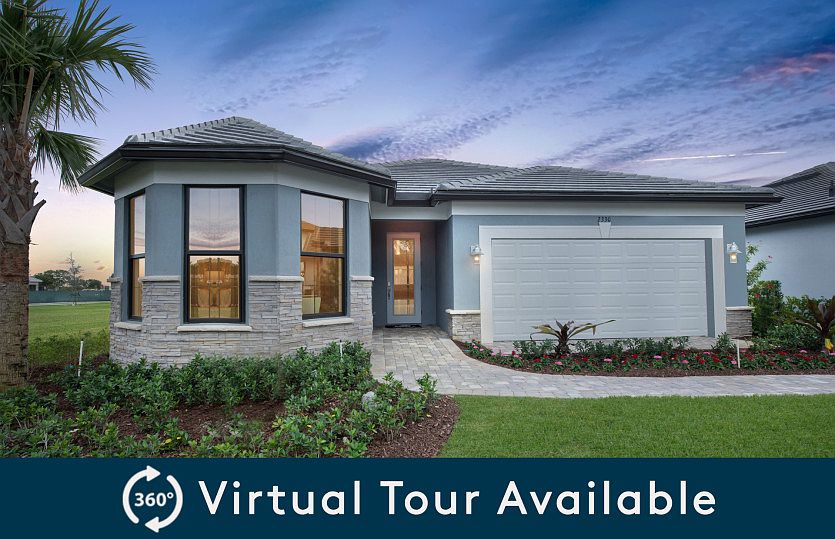This is an advertisement featuring an image of a house at sunset, set against a sky that transitions from light blue to dark blue and pink. The bottom of the advertisement has a dark blue bar with white text that reads "360-degree virtual tour available" and includes arrows pointing in each direction. The house itself is light blue with a gray tiled roof and light gray brickwork at the base. A brick pathway in matching light gray runs from the front door, located centrally, to the right side of the house.

The left side of the house features an octagon-shaped room and a small, well-manicured garden in the front left corner, accompanied by a tree. In the middle of the photo, the front door is prominently displayed, and to its right, there's a two-car garage with a white door. Another small garden area with brown and green plants is situated next to the garage, which also has two lit lights on either side. In the background, you can catch a glimpse of another light blue house on the right side.